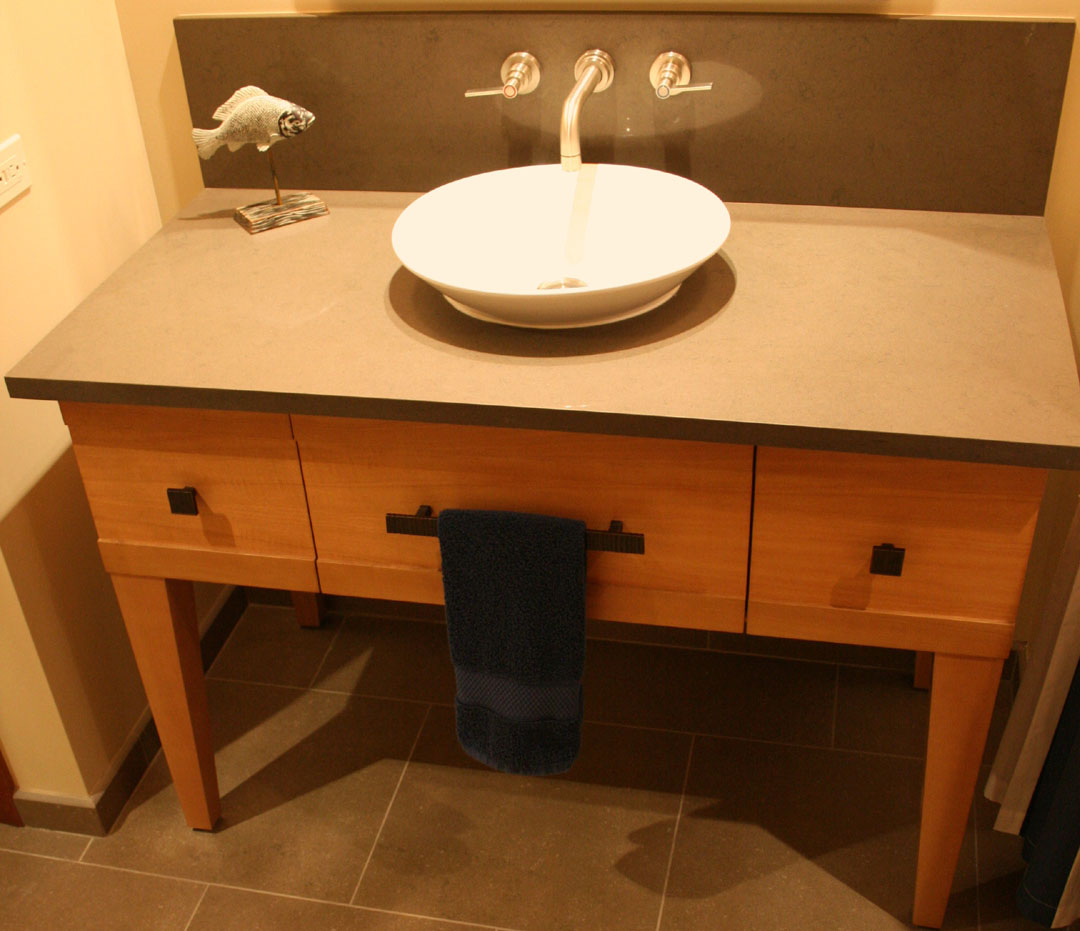This photograph showcases a beautifully crafted bathroom counter. The counter, supported by four sturdy wooden legs, features a sleek and modern design. On the front side of the counter, there are three drawers, two of which are square-shaped with black, square knobs, allowing for easy access. The middle drawer is uniquely designed with an integrated towel rack, from which a black towel is currently hanging.

The countertop is a sophisticated grayish-slate color, providing an elegant contrast to the white, bowl-shaped sink that sits atop it. The sink itself is a striking, standalone piece, adding a contemporary touch to the setup. The backsplash of the counter is equipped with a minimalist, silver-colored faucet and temperature controls, emphasizing the modern aesthetic.

Adding to the counter's charm is a small fish sculpture positioned on the left-hand side. This decorative item consists of a piece of wood with a pin holding a silver fish, giving an artistic flair to the space. The photograph overall hints that this setup is either a newly assembled bathroom counter ready to be showcased or potentially up for sale, highlighting its stylish and functional design.